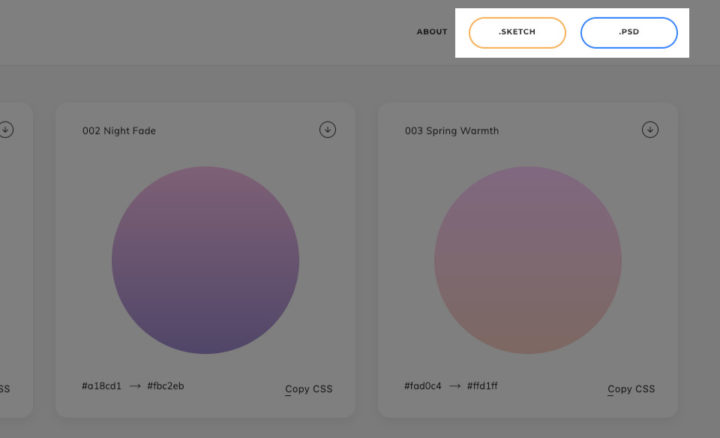Here is a cleaned-up and detailed caption for the image:

---
This image is a screenshot with a grayed-out but still visible background. In the top right corner, a prominent white rectangle stands out. Inside this rectangle, there's an orange-outlined oval labeled ".sketch" and a blue-outlined oval labeled ".psd." Just to the left of the white rectangle in the grayed-out background, two large white squares are visible.

The first white square is labeled "002 Night Fade." Inside the square, there is a deep lavender-colored circle. At the bottom of this square, text displays the color codes "#018CD1" and "#FBC2EB" with an arrow pointing to the right between them. The phrase "copy CSS" appears, with the "C" in "copy" underlined.

The second white square is labeled "003 Spring Warmth." This square features a pink circle. Below, it lists the color codes "#FAD0C4" and "#FFD1FF" with an arrow pointing to the right between them. Similar to the first square, the phrase "copy CSS" is present, with the "C" in "copy" underlined.

The overall image is wider than it is tall, providing a clear view of these design elements and their associated information.